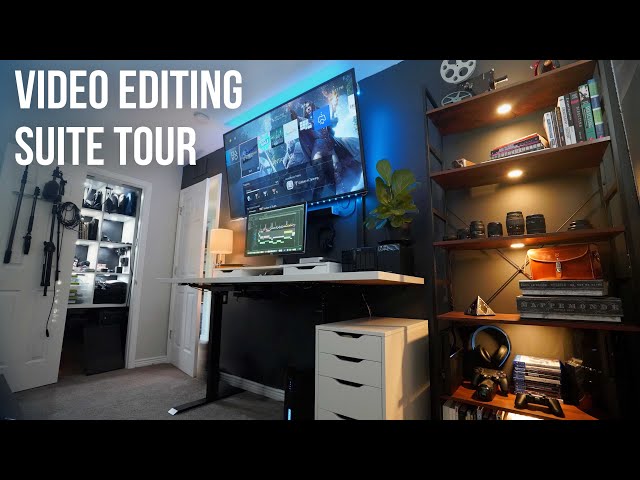The image displays a room designated as a video editing suite, prominently featuring mixed indoor elements. The primary feature is a large flat-screen TV fixed to a black accent wall, with blue backlighting enhancing its presence. Directly beneath it, a white tabletop desk supports a computer monitor, centrally poised between a lamp on the left and a green houseplant on the right. A small white filing cabinet with pull-out shelves sits below the desk. To the right of the desk, a brown bookshelf holds an assortment of books, movie reels, and stereo equipment. Adjacent to this setup is a white door, merging with the otherwise white walls of the room. Across the image, white text reads "video editing suite tour," marking the photograph. The image, taken horizontally, integrates ambient golden shelf lighting and dark room tones, contributing to an overall professional and streamlined ambiance.